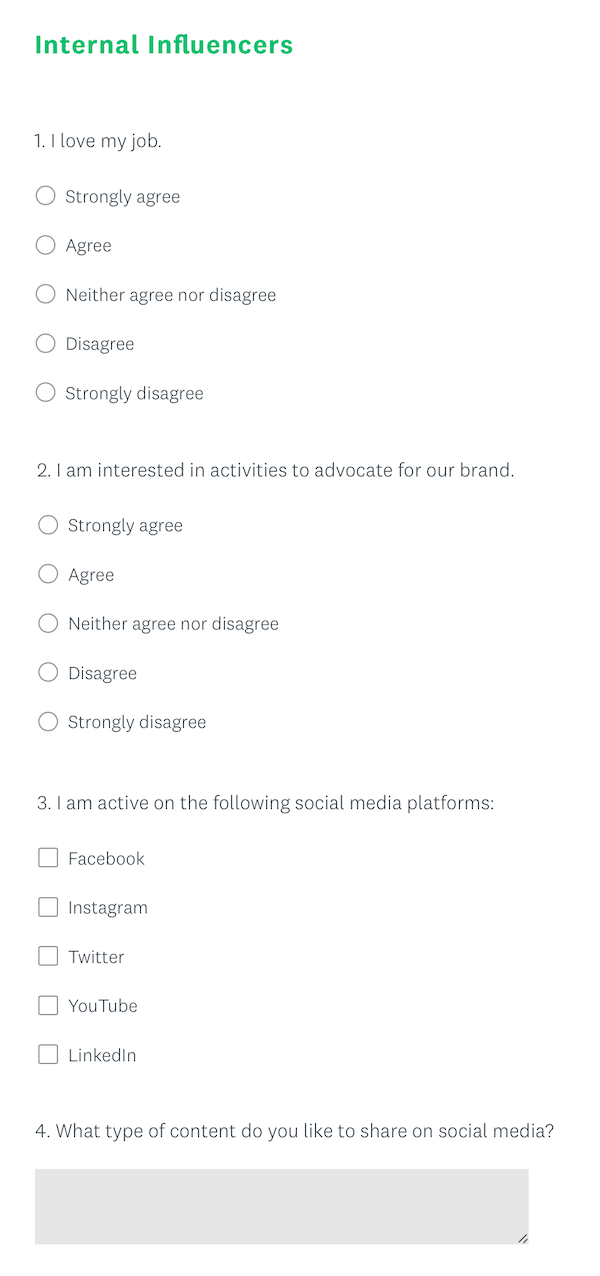This image captures a survey focusing on internal influences within a workplace, specifically assessing employee sentiments and engagement. The survey follows a structured format with multiple-choice questions.

1. **I love my job:**
   - Strongly agree
   - Agree
   - Neither agree nor disagree
   - Disagree
   - Strongly disagree

2. **I am interested in activities to advocate for our brand:**
   - Strongly agree
   - Agree
   - Neither agree nor disagree
   - Disagree
   - Strongly disagree

3. **I am active on the following social media platforms:**
   - A list of five social media platforms follows this question.

The survey is designed to gauge employee job satisfaction, willingness to support brand initiatives, and social media activity.